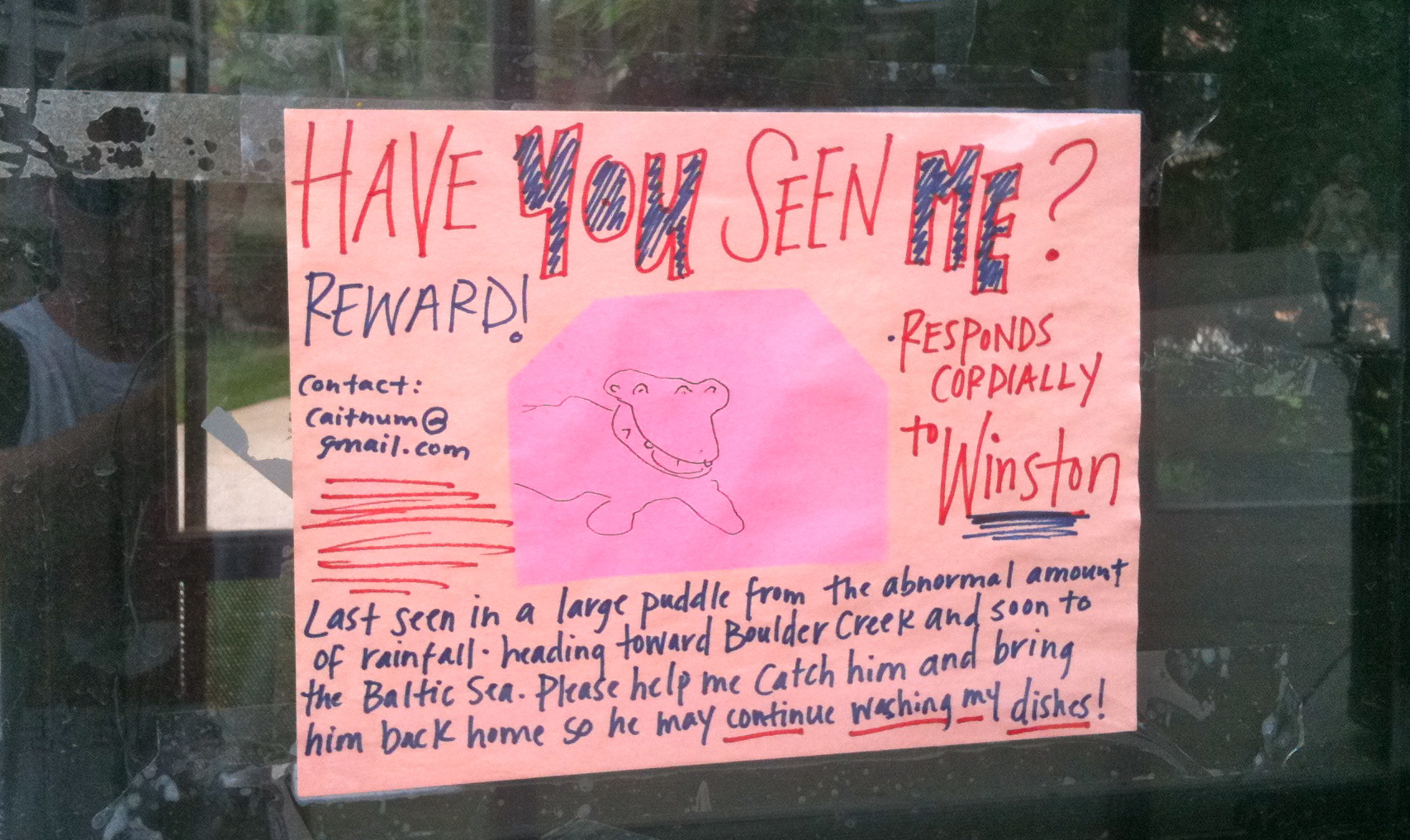The image shows a handwritten sign on a pink piece of construction paper, taped with clear tape to a highly reflective window. The window reflects an outdoor green area, and in the reflection, a woman walking on a road can be seen in the top left corner, along with a young white person, likely the one taking the photo. The pink paper has multiple lines written in marker. At the very top, in red marker with blue accents, it reads, “Have you seen me?” Below that, in blue marker, it says, “Reward!” In the center of the image, a drawing of an alligator-like creature with two eyes and an elongated mouth is enclosed in a pink hexagon. To the right of the drawing, in red marker, it reads, “Respond cordially to Winston,” with “Winston” heavily underlined in blue marker. On the left side, it says in blue marker, “Contact catenum at gmail.com,” with “gmail.com” heavily underlined in red marker. Additionally, a paragraph below the image, written in blue marker, describes the creature as last seen in a large puddle due to heavy rainfall, moving towards Boulder Creek and possibly the Baltic Sea, pleading for help to bring him back home to continue washing dishes. The overall style combines a child-like drawing with more sophisticated handwriting, suggesting a playful yet serious tone.